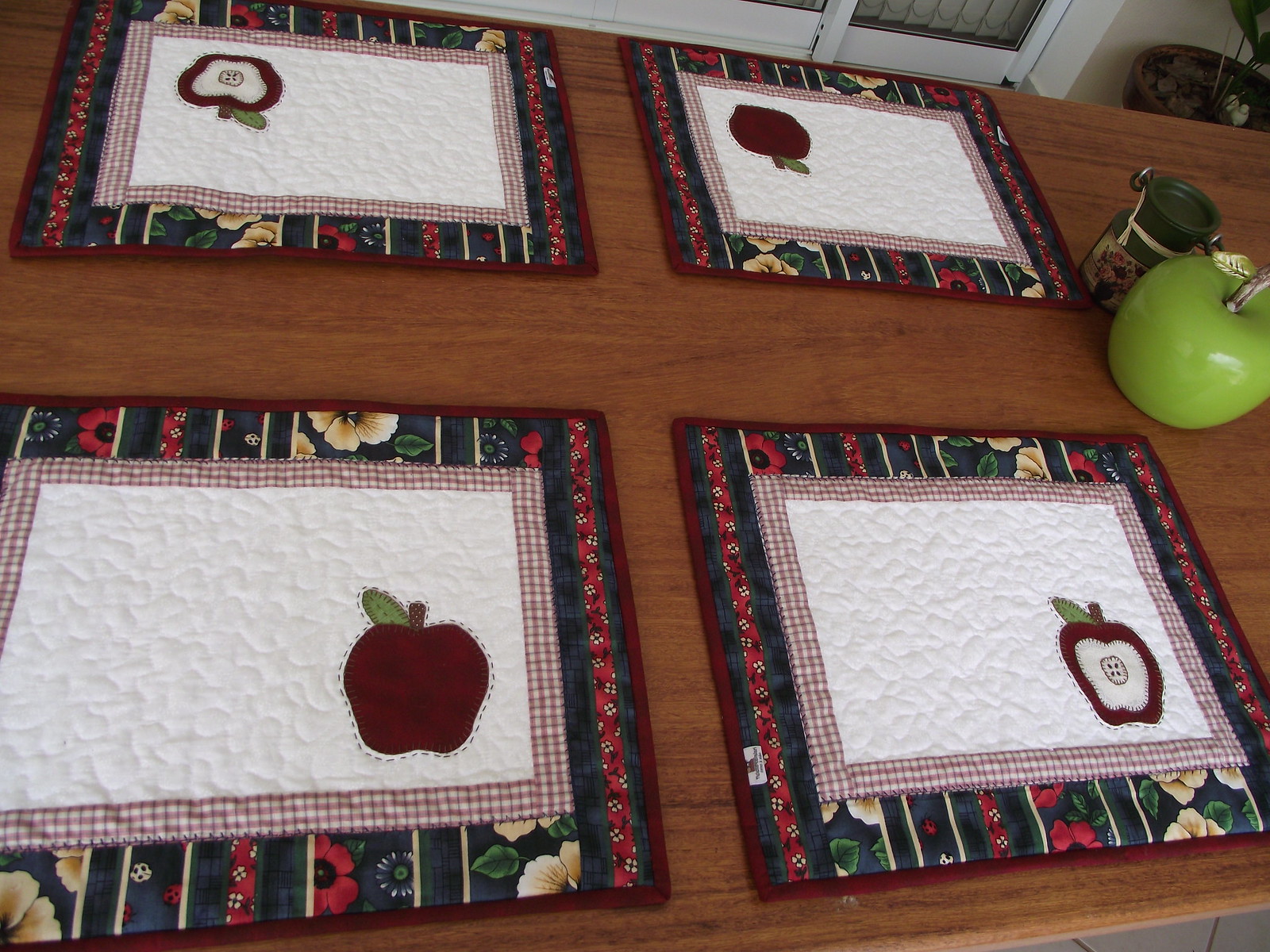This detailed photograph captures a wooden table adorned with four white-centered, hand-quilted placemats. Each placemat prominently features an apple in the lower right corner; two apples are whole and two are cut in half, revealing their white interiors. All the apples are vividly red with green leaves. The placemats boast a festive trim of red, white, and green floral, lending a Christmassy feel to the setting. Notably, the two upper placemats have their apple designs oriented upside down. On the right side of the table, a green ceramic apple with a golden leaf and a small green jar with a floral label complete the arrangement, adding an extra touch of charm.